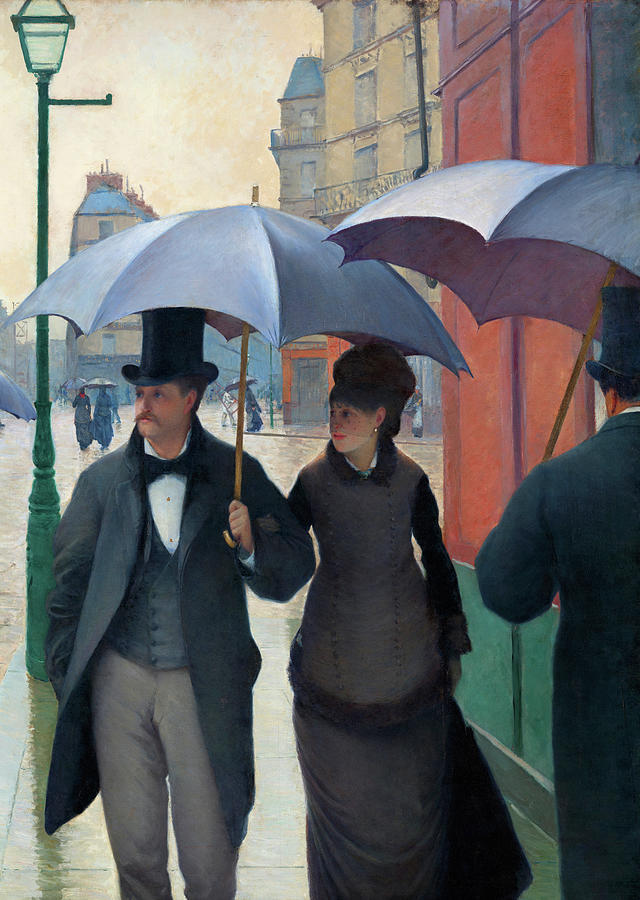This detailed painting, executed in a realistic style and possibly evoking an older European cityscape, portrays a man and a woman dressed in mid-19th century attire. The man, sporting a top hat, a white dress shirt, a black bow tie, a waistcoat, a black coat, and tan-gray pants, walks alongside the woman who is elegantly clad in a long-sleeved outfit with a white collar and a flared skirt. She is adorned with simple round pearl earrings and has her hair neatly packed atop her head. They share a large blue umbrella with a tan stem as they walk, with the woman's arm tucked under the man's. Both are looking off to the left towards something outside the frame, seemingly unaware of another man, partially cropped out and facing away, who is also wearing a top hat and holding his own umbrella.

The setting suggests a dreary day on the verge of rain, with a sky rendered in an orangish-tan hue adding to the somber mood. In the background, more people can be seen, many of whom are also holding umbrellas. The city is characterized by several tall, older buildings. Prominent among them is a bright orangish-red building with a green base situated to the right of the couple, while other buildings are mostly tan and brown, possibly serving as hotels or other establishments. A green lamppost, unlit due to the daytime setting, stands in the background to the left, further adding to the historic atmosphere of the scene.